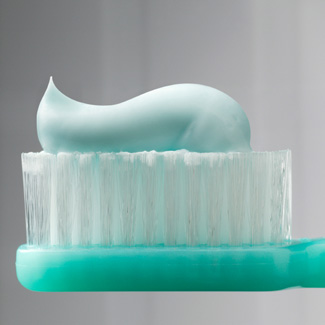A vivid square color photograph showcases an up-close view of a toothbrush head. The handle of the mint green plastic toothbrush extends from the right side of the frame. Positioned with bristles pointing straight up, the toothbrush lays flat on its plastic side, catching abundant light on its left edge. The white bristles are neatly crowned with a dollop of toothpaste, artfully swirled to resemble a soft-serve ice cream cone. The toothpaste itself is a delicate shade of light mint green, smoothly spanning nearly the entire length of the bristles.